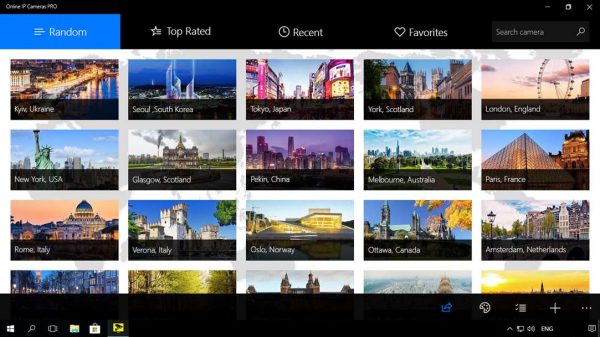A screenshot from an online website displays a grid of tiled images, each representing a different major city from around the world. The images prominently showcase famous landmarks associated with these cities, capturing their unique cultural and architectural essence. At the top of the webpage, there are several navigation options including "Random," "Top Rated," and "Recent Favorites," as well as a search bar that enables users to search for specific cameras located in various cities. A black bar at the bottom of the screen, indicative of a Windows PC interface, features several icons: the Windows logo, a search icon, a file management icon, a share button, an add images button, and an edit button. These functional icons allow the user to interact with the content on the page, providing options to share, manage, and customize the displayed images.